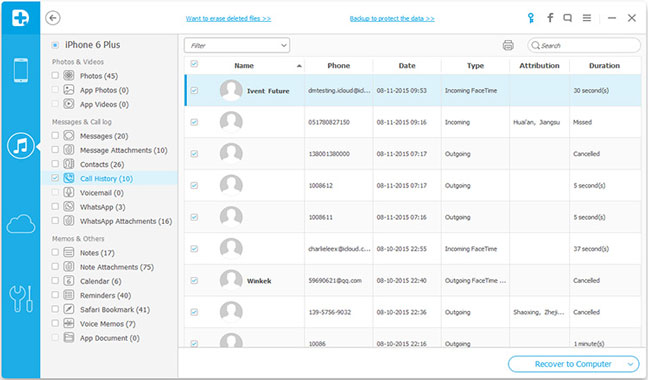The image depicts a screenshot taken from a desktop computer interface, set against a white background. On the left side of the screenshot, there is a vertical blue band containing several white-painted icons representing different functionalities: a phone logo, a music note, a cloud, and tools. The music icon is currently selected.

The main interface displays details from an iPhone 6 Plus. Various categories are listed, including "Photos and Videos," which shows the number of items in that category, "Messages and Call Logs," "Memos and Others," encompassing notes, attachments, calendar entries, reminders, and more.

Within the "Messages and Call Logs" section, the "Call History" is highlighted in blue, drawing attention to the details listed on the right side of the screen. The call history information includes the names and phone numbers of contacts, the dates of the calls, call types (outgoing or incoming), and the durations of the calls.

At the bottom of the interface, a blue text button reads "Recovered to computer."